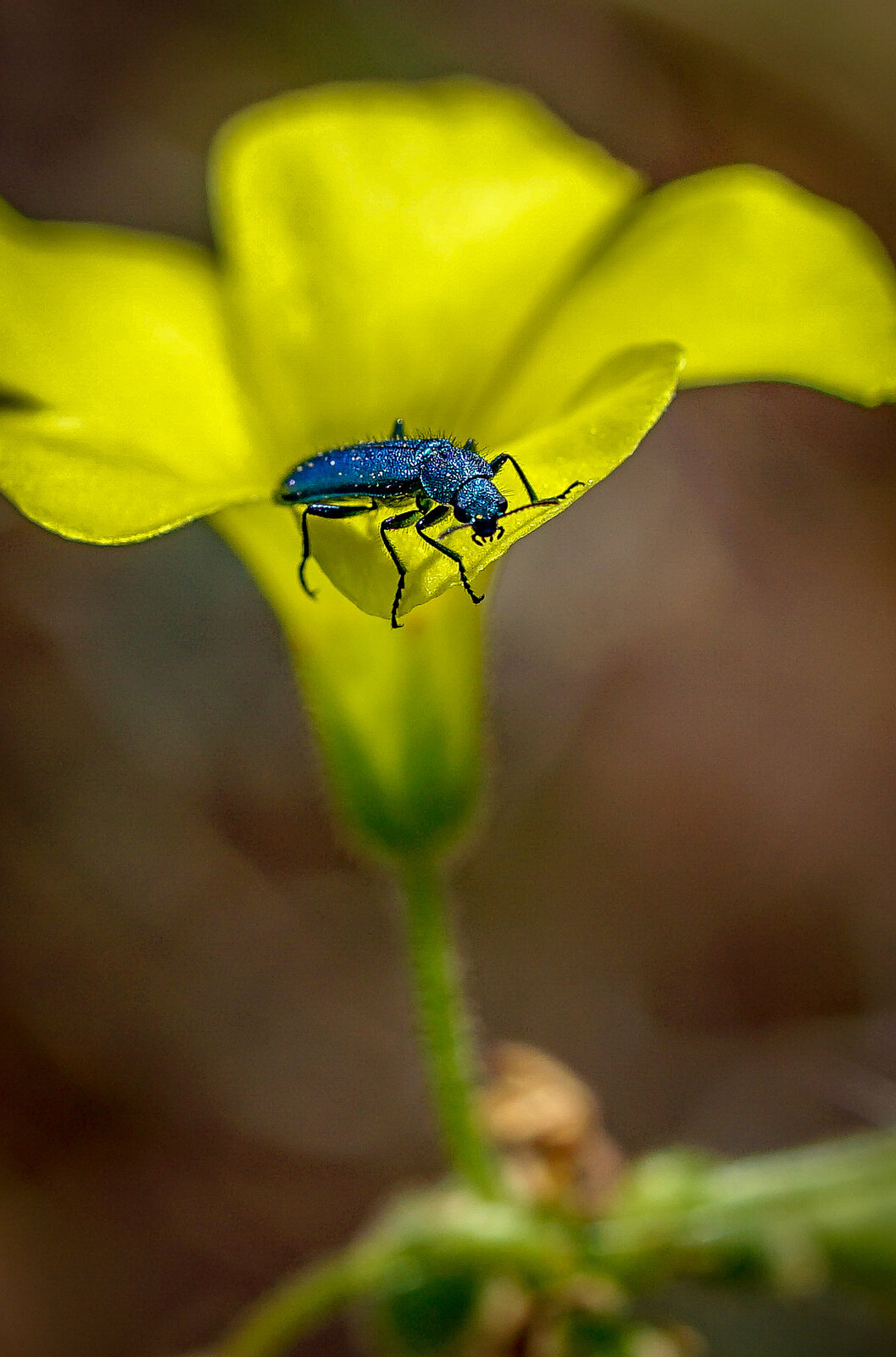This image was taken outside, featuring a striking yellow trumpet-style flower with five petals. The petals fan out at the top, creating a large, open bloom that draws the eye immediately. Perched prominently on the petal closest to the viewer is a vibrant blue iridescent beetle. The beetle’s body is adorned with tiny water droplets or possibly fuzz, adding to its textured appearance. Its six legs are black, with the front legs slightly dangling off the petal as if it's gazing towards the camera with its black beady eyes and delicate pincers. The background of the photo is a soft peachy tan that blends into brownish and whitish tones, but remains blurred to keep the focus on the flower and beetle. Additionally, some blurred green foliage and vine details can be observed, contributing to the overall natural setting of this captivating scene.